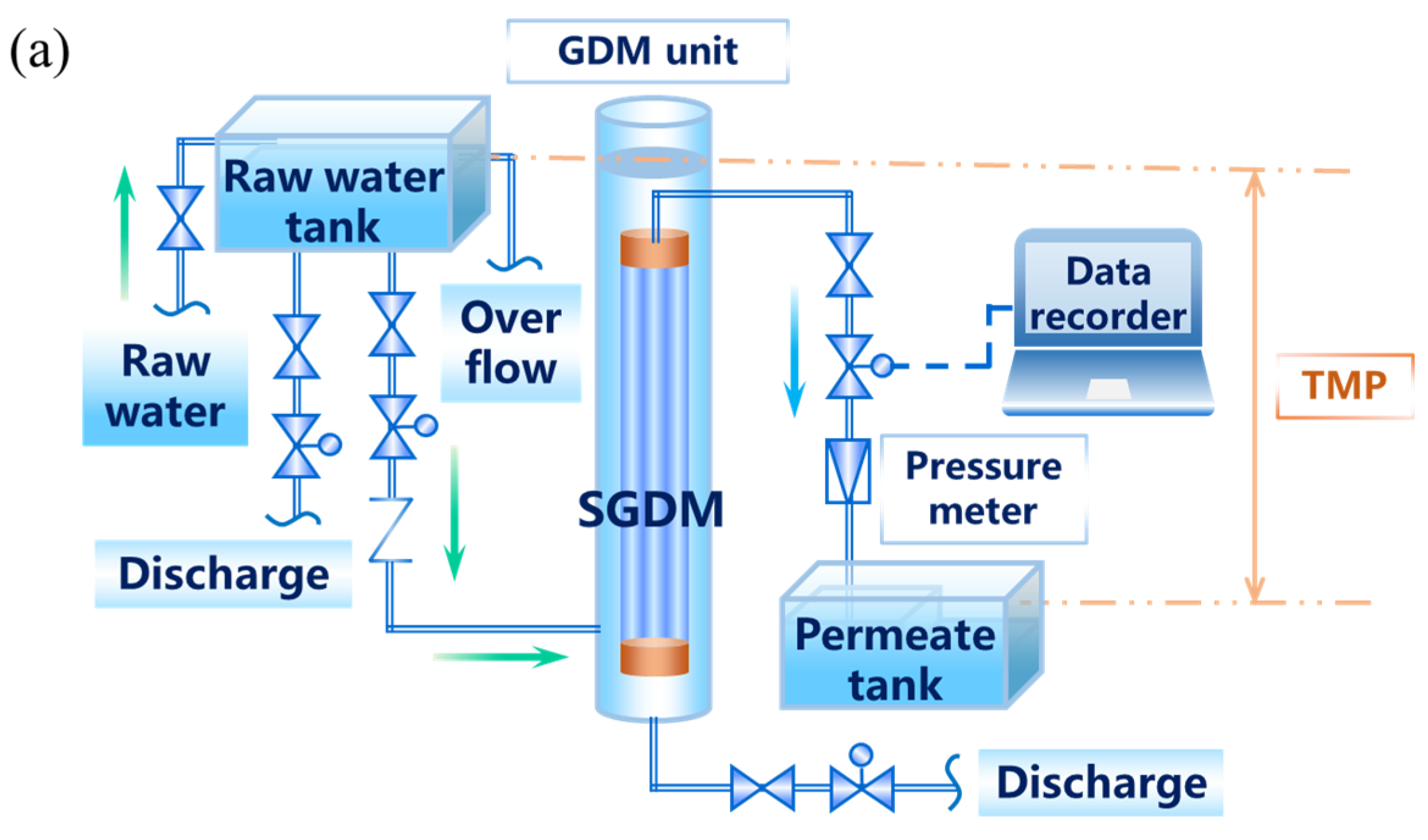The diagram depicts a GDM unit, clearly outlining the flow and treatment of water within the system. Set against a white background, it features various components indicated by labels and arrows that trace the path of water flow. In the top left corner, there are brackets around the letter 'A', while the top center prominently displays the label "GDM unit". To the left, the diagram shows a raw water tank, complete with sections for raw water, discharge, and overflow.

In the center, a large cylindrical component labeled "SGDM" signifies the main processing unit, with arrows illustrating the water's journey through the system. On the right-hand side, several key components are labeled, including a data recorder that resembles a laptop, TMP, a pressure meter, and a permeate tank. The diagram extends further right to indicate discharge points.

The entire diagram is rendered primarily in two shades of blue—light and dark—with additional highlights in orange and green. The label "DMP" stands out in orange, differing from the mostly black text used for other components, yet its significance remains unclear from the illustration. The visual aids, such as photos or depictions accompanying the labels, contribute to the clarity and comprehensibility of the flow chart. Overall, the diagram effectively presents a detailed and organized overview of the GDM unit and its various parts.